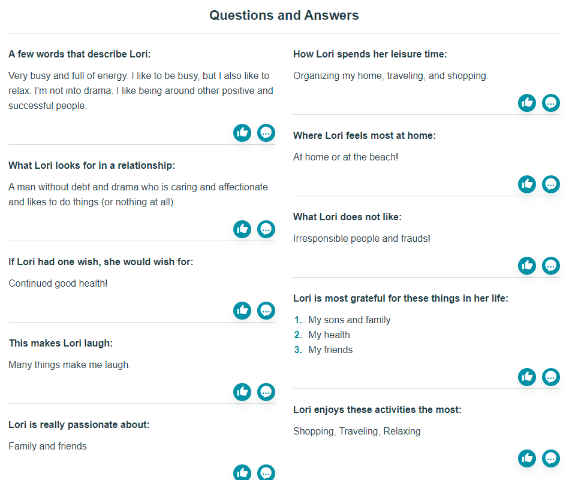In the center of the image, there is a bold, black heading that reads "Questions and Answers." A thin line separates various sections. To the left, there is a tile without an outline containing a few words that describe Lori: "very busy and full of energy." Below this, the text elaborates, stating, "I like to be busy but I also like to relax. I'm not into drama. I enjoy being around other people, especially successful individuals." To the right, there are thumbs up and comment buttons. 

Another line follows and introduces what Lori looks for in a relationship: "a man without debt and drama who is caring and affectionate and enjoys doing things, or nothing at all." Again, there are thumbs up and comment buttons below. Following another line, it reads: "If Lori had one wish, she would wish for continued good health." The same buttons are present beneath this section. 

Continuing, another line leads to the text: "This makes Lori laugh: Many things make me laugh," followed by the familiar thumbs up and comment buttons. Another line then describes what Lori is passionate about: "family and friends."

Returning to the top on the right side, the text describes how Lori spends her leisure time: "organizing my home, traveling, and shopping," followed by the familiar two buttons. Another line follows, describing where Lori feels most at home: "at home or at the beach," with the same two buttons below it.

The remaining three sections, separated by lines, state:
- "What Lori does not like"
- "What Lori is most grateful for"
- "The activities Lori enjoys"

Each section continues the pattern of including thumbs up and comment buttons.